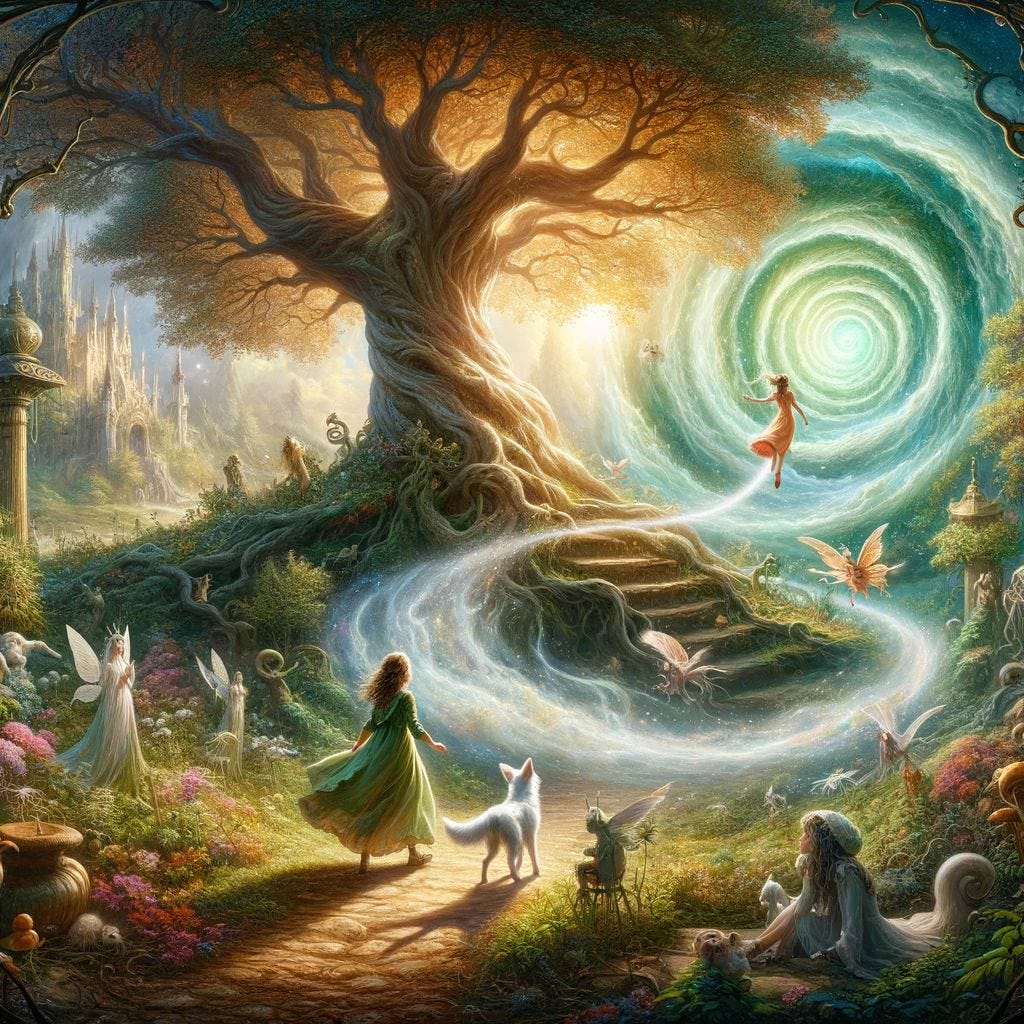In this richly detailed fantasy painting, a sprawling, massive tree dominates the scene, its colossal trunk adorned with countless roots and knots. The tree’s foliage, a vivid burst of orange, suggests a vibrant fall setting. Intricate wooden stairs seamlessly integrated into the tree’s structure spiral upwards, inviting exploration. To the left, a majestic white castle stands with numerous spires reaching skyward, adding a regal touch to the landscape.

Amidst the enchanting scenery, various fairy queens flit about, their delicate white wings shimmering against their elegant crowns and flowing dresses. A woman, draped in a lush green cloak and dress, stands confidently on a brown brick path, accompanied by her faithful white dog.

Nearby, another woman in a white gown sits serenely, affectionately petting a mystical creature. Additional fairies in hues of white and orange add to the ethereal atmosphere, their details less discernible but still magical. 

To the right, a particularly striking scene unfolds as a woman in an orange dress, surrounded by an aura of white magic, ascends into a swirling green vortex. This magical gateway, filled with clouds and mystery, hints at an otherworldly destination. The entire scene melds together to form a captivating tableau of an enchanting fantasy realm, filled with enchanting beings, majestic trees, and mysterious portals.